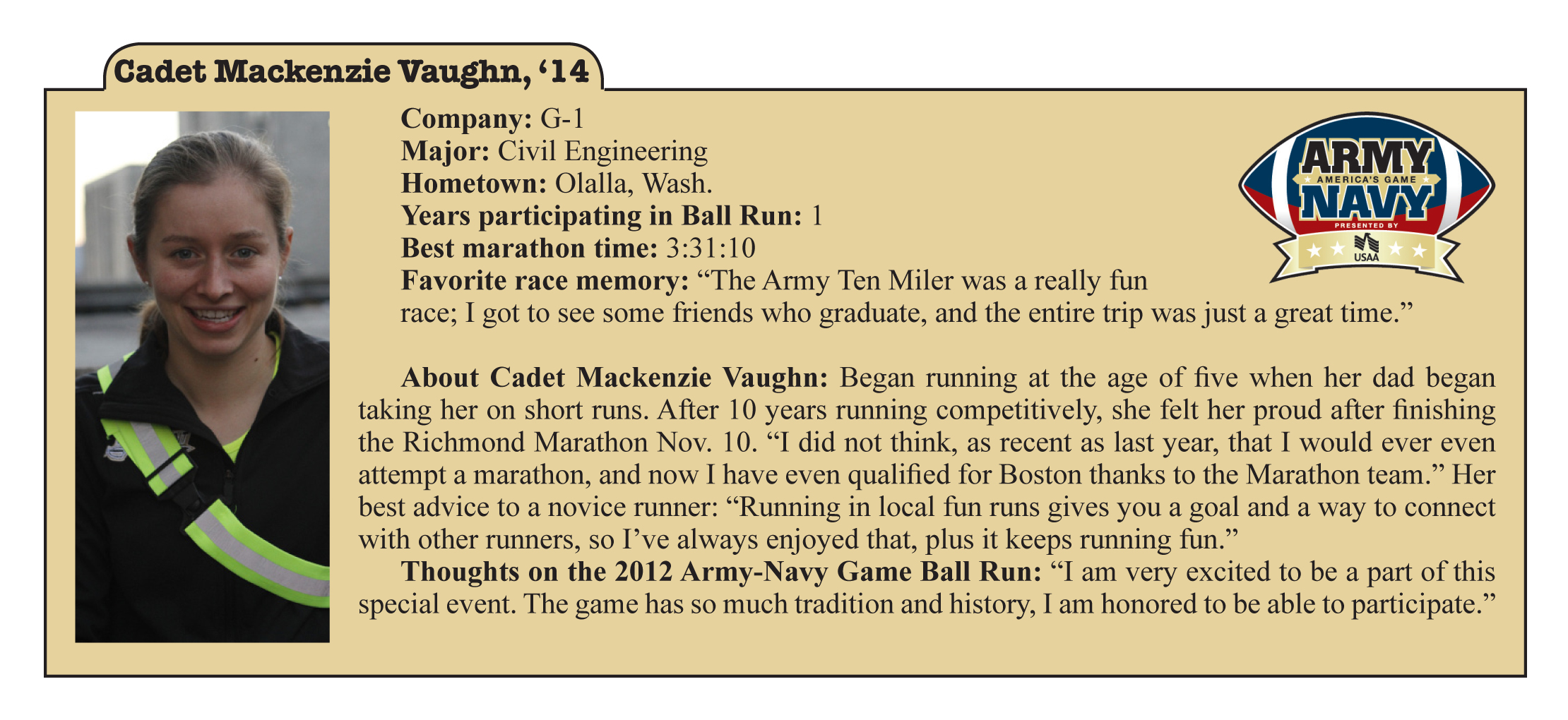The image is a detailed informational piece featuring Cadet McKenzie Vaughn set against a yellow background with black text. In the top left corner, a yellow rectangle contains the information: "Cadet McKenzie Vaughn, class of 2014, Company G-1," with her major listed as civil engineering. The text also notes her hometown, Ola, Washington. Years participating in the ball run: one. Best marathon time: 03:31:10. Her favorite race memory is the Army Ten-Miler, where she enjoyed seeing friends graduate and had a great trip overall.

The top right corner displays a blue and red football with the text "Army vs. Navy" and a small, presumably unreadable text, along with a ribbon below that says "USAA" with stars on either side. Additionally, there are two more sections providing details about McKenzie. A portrait of McKenzie Vaughn, a blonde Caucasian woman in uniform, accompanies the text.

Further details on McKenzie include her starting to run at the age of five with her dad. She boasts over ten years of competitive running, with a notable achievement of finishing the Richmond Marathon on November 10th. She expressed pride in qualifying for the Boston Marathon with the help of her marathon team, despite never having thought she would attempt a marathon as recently as the previous year. McKenzie’s best advice for novice runners is to participate in local fun runs to set goals and connect with others, which makes running enjoyable. Reflecting on the 2012 Army-Navy game ball run, she feels honored to partake in an event rich in tradition and history.